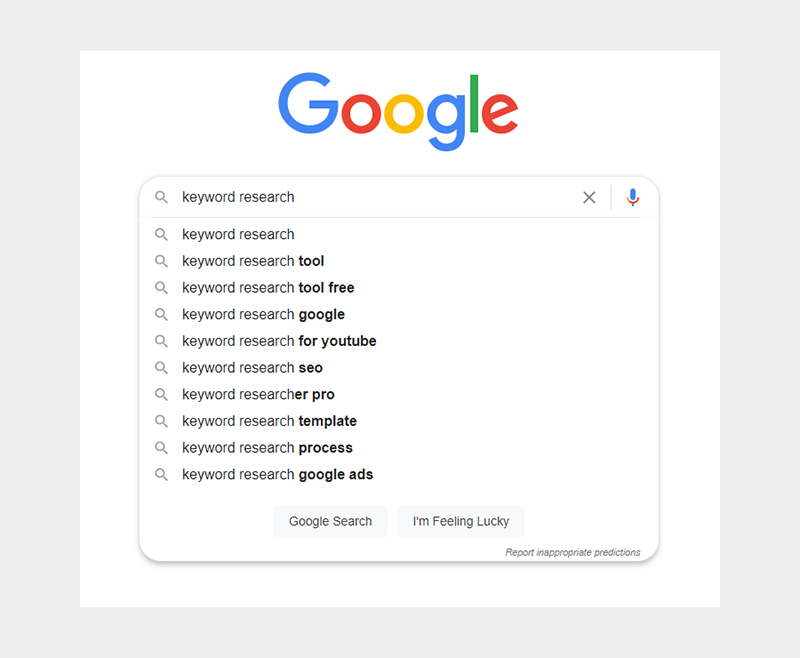The image is a screenshot from a website with a light gray background that is thicker on the left and right sides. The main content is centered within a white square. At the top of the square, the Google logo is displayed, featuring multi-colored letters: a blue 'G', red 'o', yellow 'o', blue 'g', green 'l', and red 'e'.

Below the logo is a search bar, accompanied by a magnifying glass icon on the left and a blue "X" on the right, signifying the option to clear the search text. To the right of the "X" is a microphone icon, indicating voice search capability.

Inside the search bar, the text "keyword research" is typed. Directly beneath, there are suggestions for related searches listed progressively:

1. Keyword research
2. Keyword research tool
3. Keyword research tool free
4. Keyword research Google
5. Keyword research for YouTube
6. Keyword research SEO
7. Keyword research Pro
8. Keyword research template
9. Keyword research process
10. Keyword research Google Ads

These suggestions are highlighted in a darker font to differentiate from the background.

At the bottom of the white square are two buttons: "Google Search" and "I'm Feeling Lucky", inviting the user to initiate the search or try their luck with a random relevant webpage respectively.